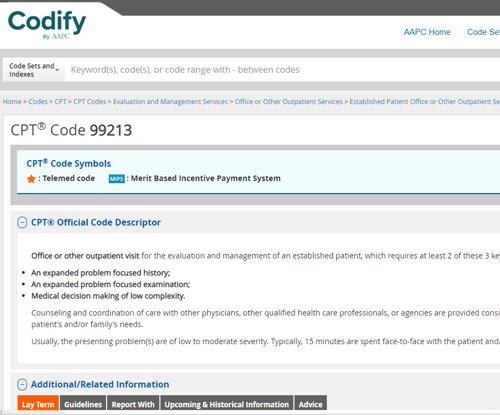This is a cropped screenshot showcasing a section of the Codify by AAPC website. The image captures the top left corner of the webpage, excluding the browser bar and most of the page. The webpage features a clean, white background. Prominently displayed at the upper left corner is the "Codify by AAPC" logo. Adjacent to the logo, centered vertically, is a blue link labeled "AAPC Home." Below this link, partially cut off, is another word that does not appear in full.

Further down, there is a horizontal banner with a grey background. On the banner's left side is a drop-down menu labeled "Code Sets and Indexes." To the right of the drop-down menu is a search bar designed for entering keywords, codes, or code ranges, indicated by placeholder text in grey.

Immediately below the grey banner is a lighter grey navigation strip. This strip includes breadcrumb links such as "Home," "Codes," "CPT," followed by "CPT Codes." Below this navigation strip is a display area introducing "CPT Code 99213," accompanied by relevant code symbols and descriptors detailing the code's specifics.